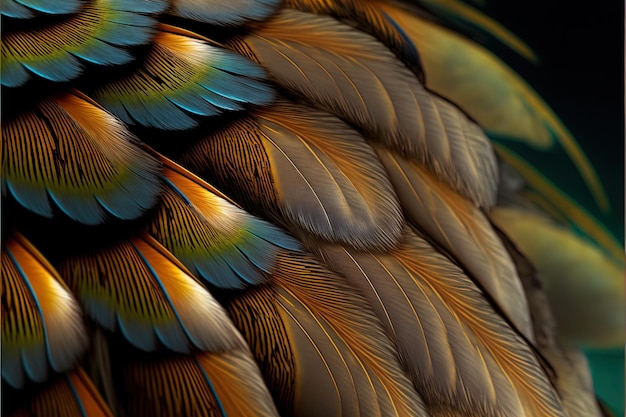This is a highly detailed, digitally created or computer-generated image of an extreme close-up of a bird's feathers, showcasing intricate patterns and vibrant colors. The composition features two sets of feathers, each with distinctive color palettes and textures. One set displays bright hues of blue, yellow, orange, and a hint of green, while the other set includes light brown, gray, and orange feathers. The feathers are layered and exhibit a mix of short, fluffy textures and long, soft strands. Iridescent blue tips gleam on the feathers to the left, adding a shining touch, while the feathers towards the bottom have soft, warm appearances with orange stripes down their centers. The background is a solid black, slightly blurred, which makes the vivid colors of the feathers stand out more prominently. There are no other elements such as bird heads, other animals, structures, or writing present in the image, allowing a focused appreciation of the rich, colorful texture of these feathers.